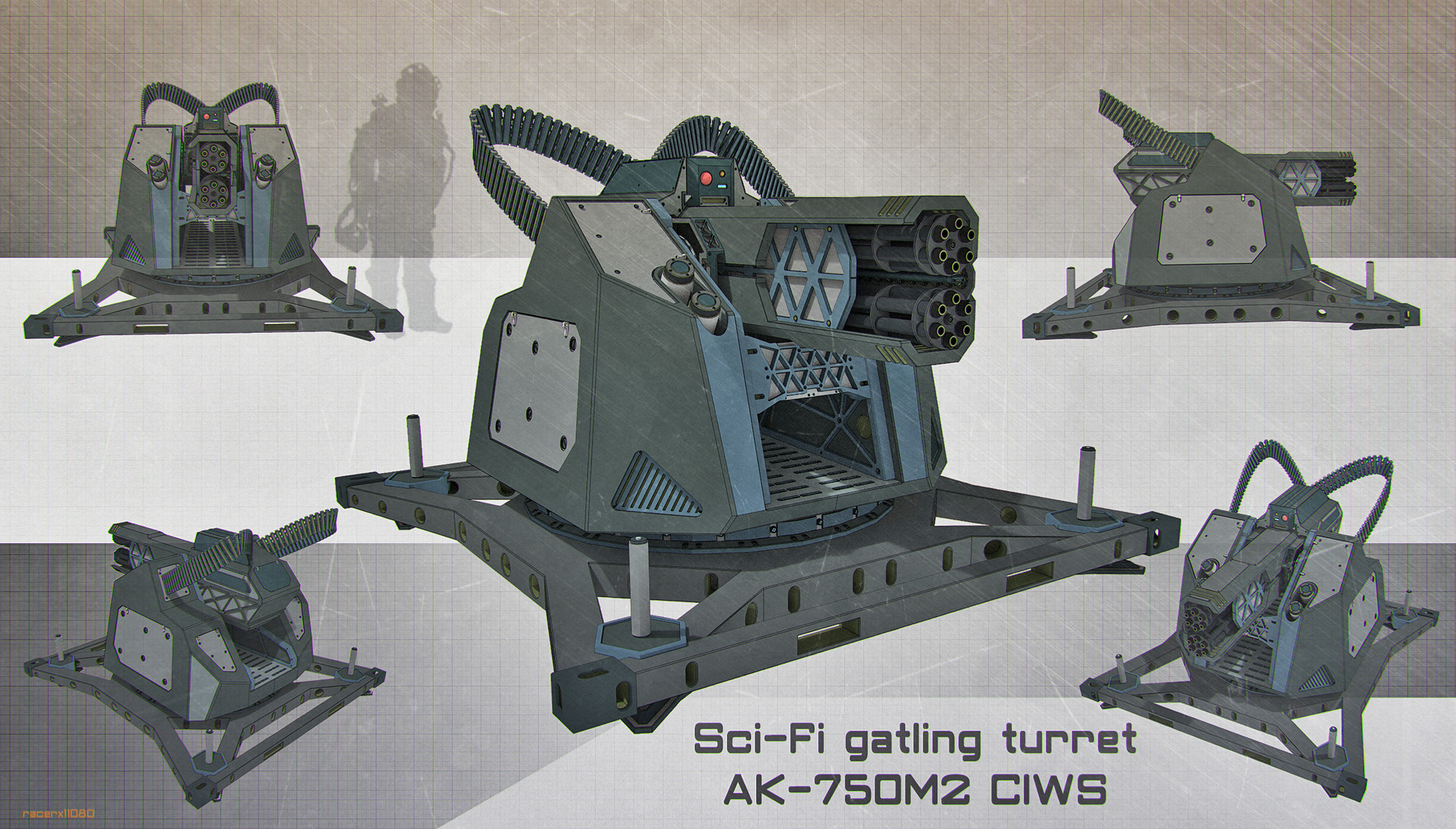The image depicts a highly detailed series of concept designs for a futuristic, automated military turret. Five different perspectives highlight the intricacies of the "Sci-Fi Gatling Turret AK-750 M2 CIWS." This turret, standing shoulder-height next to a standard-sized soldier as shown in the top-left illustration, seems particularly imposing. It features dual rotating gatling barrels, supported by two belt-fed ammunition systems, underscoring its high rate of fire. The design appears to be fully automated or possibly AI-operated, intensifying its intimidating presence. While the technology is chilling if intended for real-world military use, it’s more plausible that these designs are crafted for a video game or a television show, given their sci-fi aesthetics and warning labels.